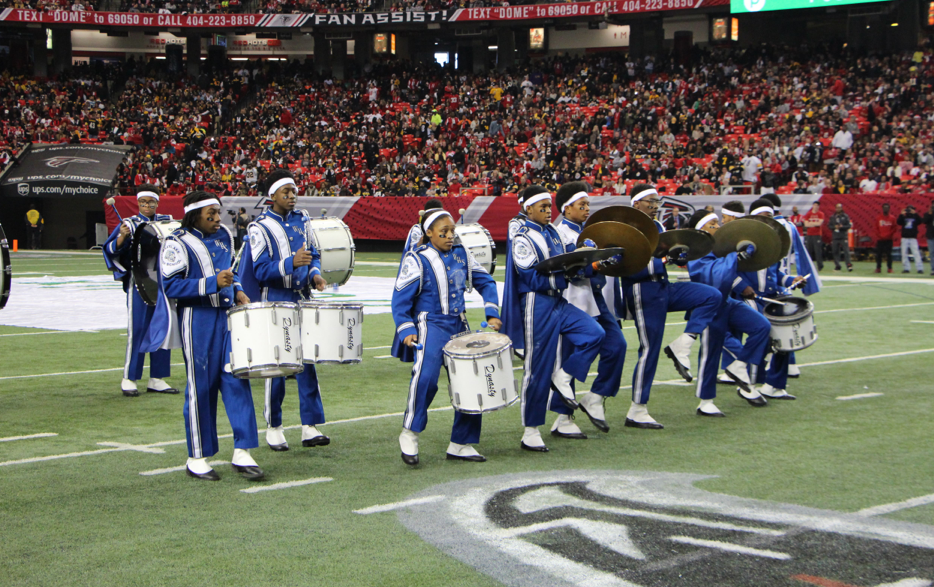This live, landscape-mode photograph captures a vibrant halftime performance on a football field. At the center of the image, approximately nine or ten African-American teenagers, male and female, are dressed in blue and white marching band uniforms, complete with white socks and black dress shoes. They are predominantly percussionists, featuring a variety of white drums, including bass and snare drums, alongside several cymbal players. Each band member has a white ribbon tied around their dark black hair, and they are seen marching towards the right side of the frame, advancing near midfield where the Atlanta Falcons logo is clearly visible.

The green grass field is neatly marked with white lines, and the sun casts a gentle light over the scene. In the backdrop, the top part of the stadium is filled with fans predominantly wearing red, with some advertisements visible, including "text DOME to 69050 or call 404-223-8850" and "ups.com/my choice." A red banner bearing the Atlanta Falcons logo adds to the festive atmosphere. The clear signage for "fan assist" and "text DOME" spans the top end of the stadium, and more advertisements can be seen scattered around. The sidelines are lined with onlookers, absorbing the engaging performance of the marching band.